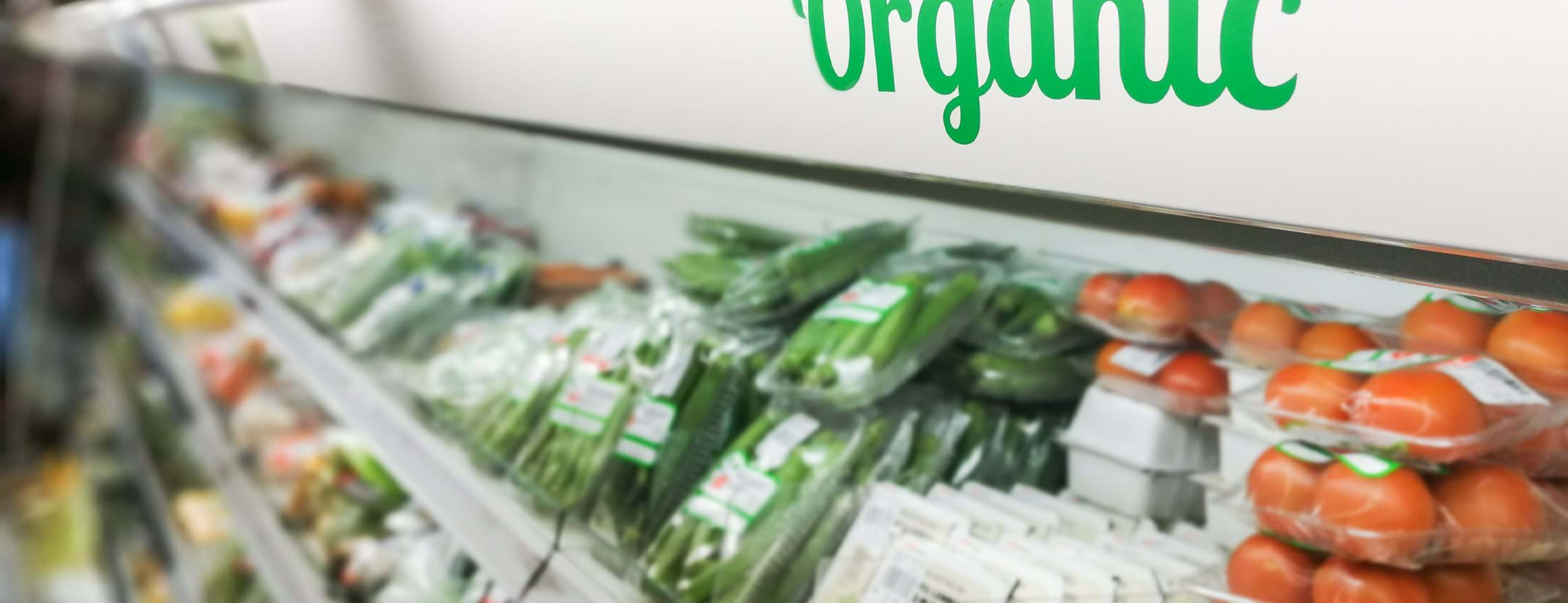The image depicts an indoor scene of a grocery store, specifically the produce section, characterized by an "Organic" label in cursive lime-green text on a white wall. The topmost shelf, closest to the viewer, displays neatly packed Roma tomatoes in clear plastic shells, exhibiting a vibrant red hue with a slight orangish tint. Adjacent to these packages are green cucumbers also encased in plastic. Below this shelf, the contents become progressively blurrier, revealing a mixture of yellows, oranges, and greens indicating various other types of produce that are indistinct but presumed to be an assortment of fresh vegetables. The shelving unit continues to hold rows of similarly packaged produce, extending into the background, but the details remain unclear due to the image's lack of focus.